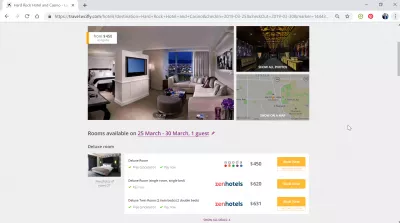The image features a gray background with a website interface displaying three distinct sections. 

- The first section showcases a photograph of a spacious hotel room. The room is well-lit with natural light streaming in through the large windows, which are adorned with drapes pulled to the sides, revealing a stunning city skyline. A flat-screen TV is mounted on the wall, and a cozy couch is positioned for relaxation.

- The second section is a dimly lit image of what appears to be the interior of a factory or industrial facility, characterized by visible machinery and a lack of natural light.

- The third section includes a detailed map with a scroll bar on the right side. The map displays information about room availability from March 20th to March 30th, indicated in purple. The section also mentions options for one guest, a small picture of a bed implying hotel room availability, and a segment dedicated to discovering reviews. There are three list items featured, and to the right of this list are three small gold rectangles with white text that is too small to read clearly.

This caption provides a comprehensive and detailed description of the complex web interface and its elements.